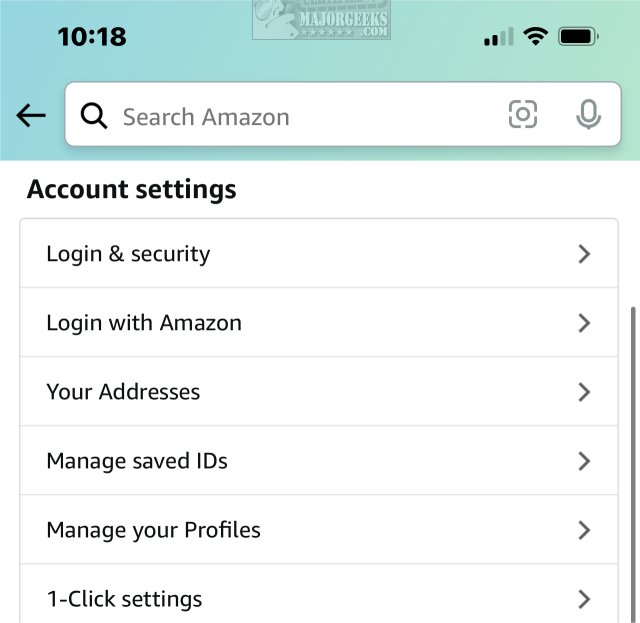This is a screenshot from an Amazon app displayed on a smartphone. At the top, the time reads 10:18. The phone shows two bars of cellular coverage, full Wi-Fi signal strength, and a fully charged battery. Below the status bar is a search bar labeled "Search Amazon." The main section of the screenshot shows various account management options including "Account Settings," "Login and Security," "Login with Amazon," "Your Addresses," "Manage Saved IDs," "Manage Your Profiles," and "1-Click Settings." Notably, no people, plants, animals, or inanimate objects like buildings or vehicles are present in the image. The screenshot includes a watermark for majorgeeks.com at the top, emphasizing that it is an illustrative and text-based image.